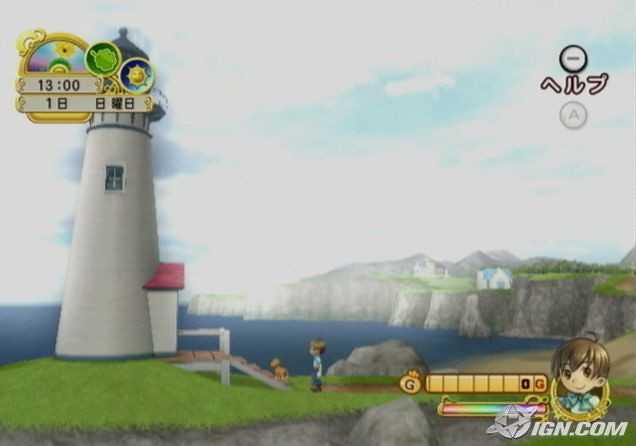The image is a detailed screenshot from a video game, stamped with an IGN watermark at the bottom right corner. The scene features a serene coastal setting with a lighthouse situated on a small, raised grassy area to the left, accessible by a set of steps leading to a platform. At the foot of these steps stands a character with short, shaggy brown hair styled with a cowlick, wearing a white shirt and a green bow around the neck. In front of this character is a small dog.

In the background, a tranquil inlet of the ocean can be seen, bordered by tall, gray cliffs that almost encircle the water. Beyond the cliffs, there are two houses; the closer one is small with a blue roof and white walls, while the larger one is set slightly farther back. Mountains loom distantly on the horizon under a sky filled with clouds, with patches of blue peeking through.

The image also features various game UI elements. At the bottom right, next to the watermark, is an anime-style portrait of a smiling boy inside a gold circle. Adjacent to the portrait, a segmented yellow bar with the letter "G" at the far left likely indicates a meter display. Below this meter, a smaller, rainbow-colored bar appears to be full. In the top left corner, the time "13:00" is shown, suggesting an in-game clock or scorekeeping mechanism. Additionally, at the top right, there is Japanese text explaining an action associated with pressing the Minus button, and below it, a grayed-out "A" button icon. 

This detailed display combines scenic elements with functional gaming interfaces to create an engaging visual experience.